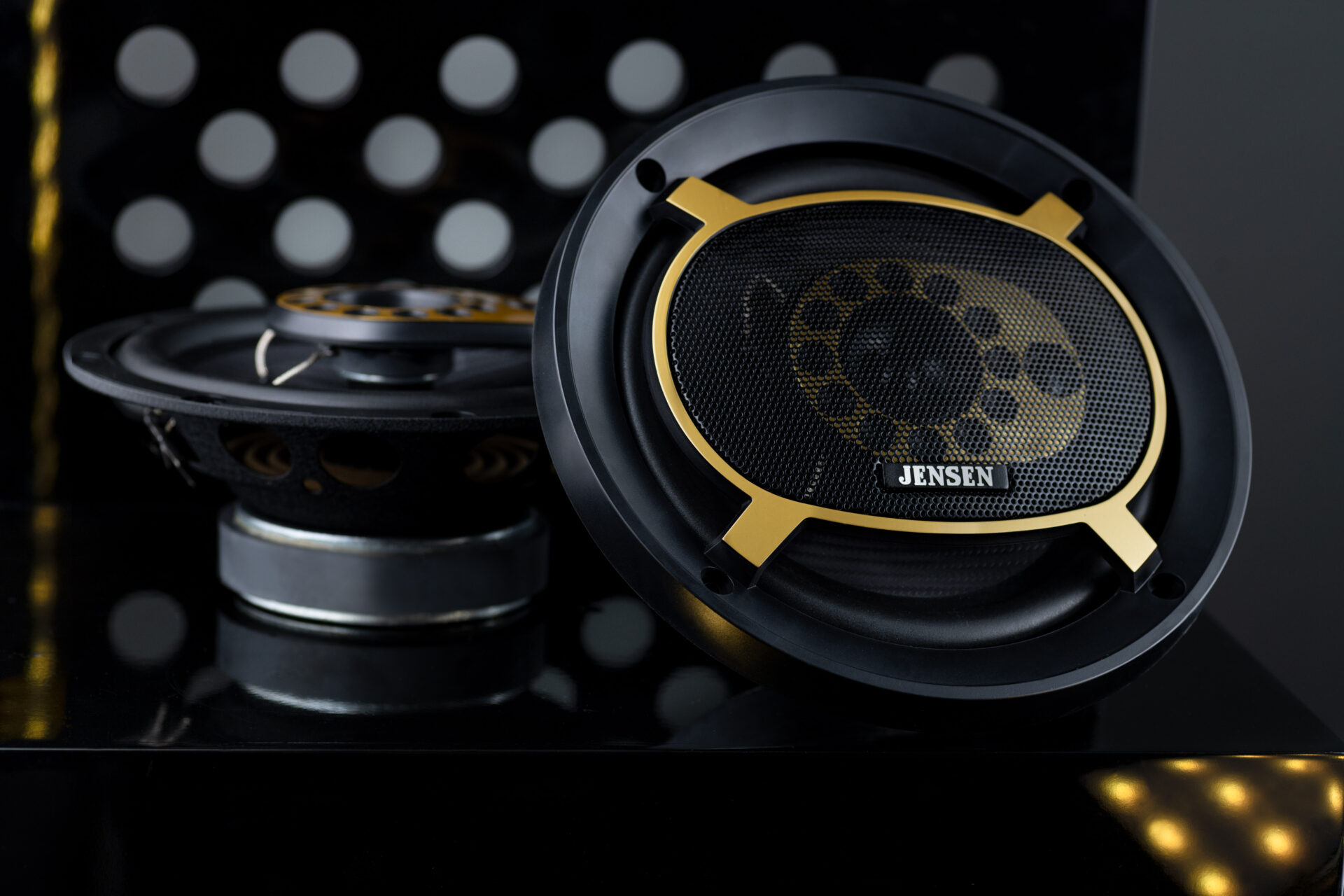This image features a pair of Jensen speakers, prominently displayed on a glossy black table against a gray background. The speaker on the left is positioned upright, showing its cylindrical side, which is adorned with a mix of black, silver, and gray colors. The speaker on the right faces the camera directly, revealing its round front. The edges of this front-facing speaker are black, transitioning to a gold interior with a black mesh screen in the center. The name "Jensen" is clearly labeled on this mesh screen. The background includes a panel with small holes and a yellow light emanating from the bottom right corner, adding a subtle glow to the scene. Overall, the image showcases the distinct colors of gold, yellow, black, silver, and various shades of gray, emphasizing the speakers' sleek design and branding.